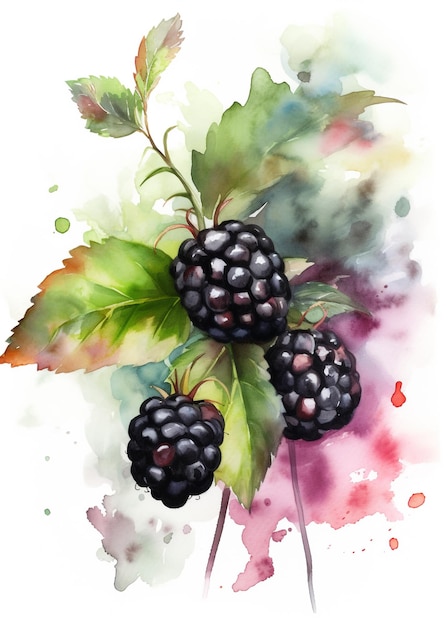This is a detailed watercolor painting of a blackberry bush, featuring three large, juicy blackberries attached to a stem with green leaves. The berries are depicted as tightly bound clusters, with a few showing touches of white on some of the individual segments. The background is a white canvas adorned with a free-form splashing of colors, predominantly purples, reds, pinks, and greens. These colors create a mottled, splatter effect reminiscent of water dripped on paper, giving the impression of a stylized, somewhat abstract scene. The overall composition suggests a natural yet artistic representation of the blackberries, making it suitable for framing or inclusion in a book.